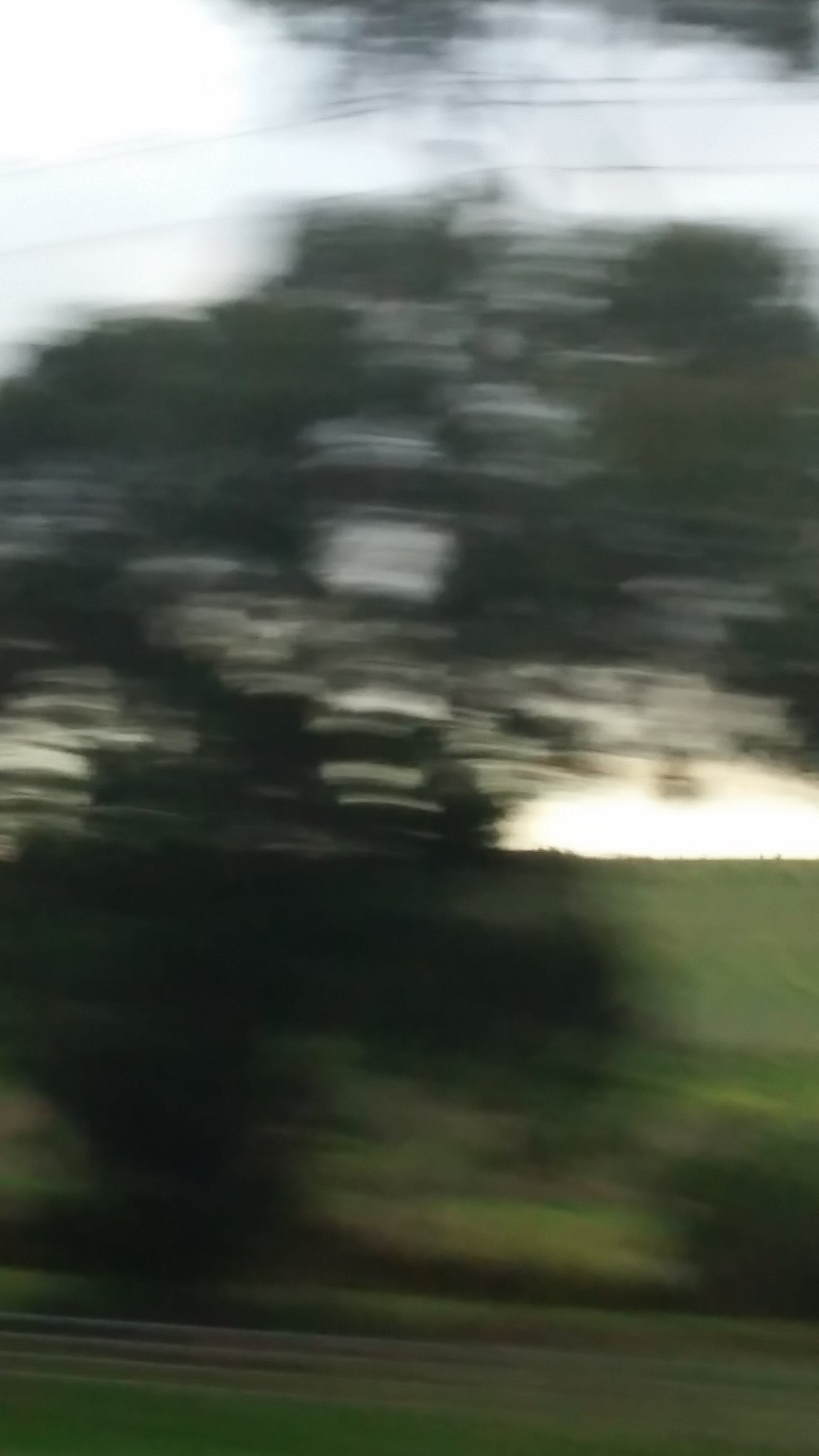This image is an extremely blurry photograph taken outdoors, possibly from a moving car, as the camera appears to have been in motion when the shutter was open. The upper portion of the image features a bluish sky with streaks of black beneath it. This black area might represent telephone lines, though they're not distinctly clear. In the central part of the image, there's a very large, tall tree that is heavily blurred, making its details indistinguishable. Below the tree, there’s a horizon line marking a field of grass which has green hues combating the blur. The photograph does not contain any people, cars, or text. The overall color palette consists mainly of different shades of green and blue, with patches of dark green, lighter green, and an area of bright white light that streaks through the middle. The right side of the image hints at a sunrise or sunset with lighter regions, further muddled by the blur. The focus remains primarily on the tree, the field, and the wide open sky.